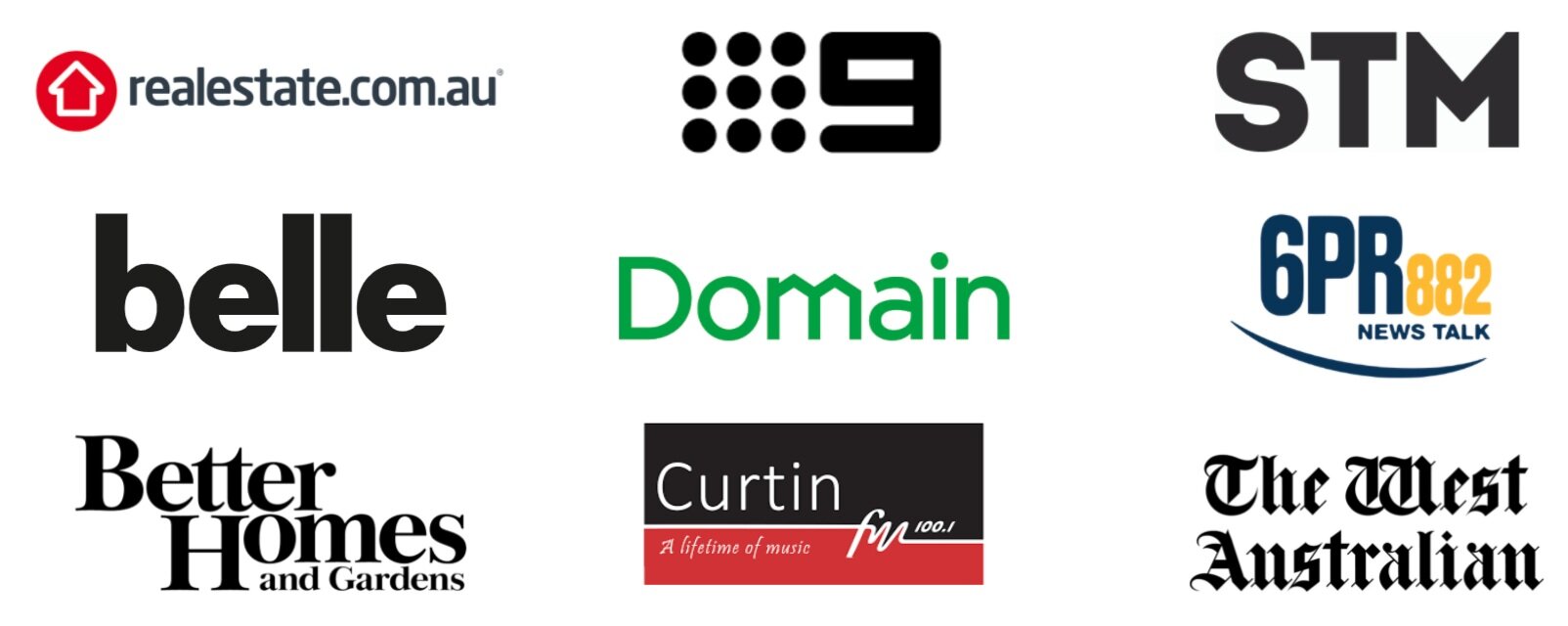This image is a screenshot of a partial web page displayed on a computer monitor, specifically from the website realestate.com.au. The top left corner of the image prominently features the logo of realestate.com.au, which is a round red circle with a white line drawing resembling a house.

Below the logo, there is a series of icons and text representing different businesses or services. Starting from the left:

1. A grid of nine black dots followed by the numeral "9".
2. The uppercase letters "STM".
3. To the bottom left, the word "belle" in lowercase letters.
4. To the right of "belle," the word "domain" in green text.
5. A sequence involving the numeral '6' followed by "PR" in uppercase letters, and the numeral "882" situated below.
6. Below "882", the term "NEWSTALK" in dark blue text with a dark blue swoosh beneath it. 

Following this sequence, rightward:

7. The well-known "Better Homes and Gardens" logo and text.
8. The label "CURTIN FM 100.1, A Lifetime of Music" to the right.
9. Finally, the label "The West Australian" concludes the series.

Each of these elements represents different entities or media organizations, distinguished by their unique logos, colors, and textual representations.